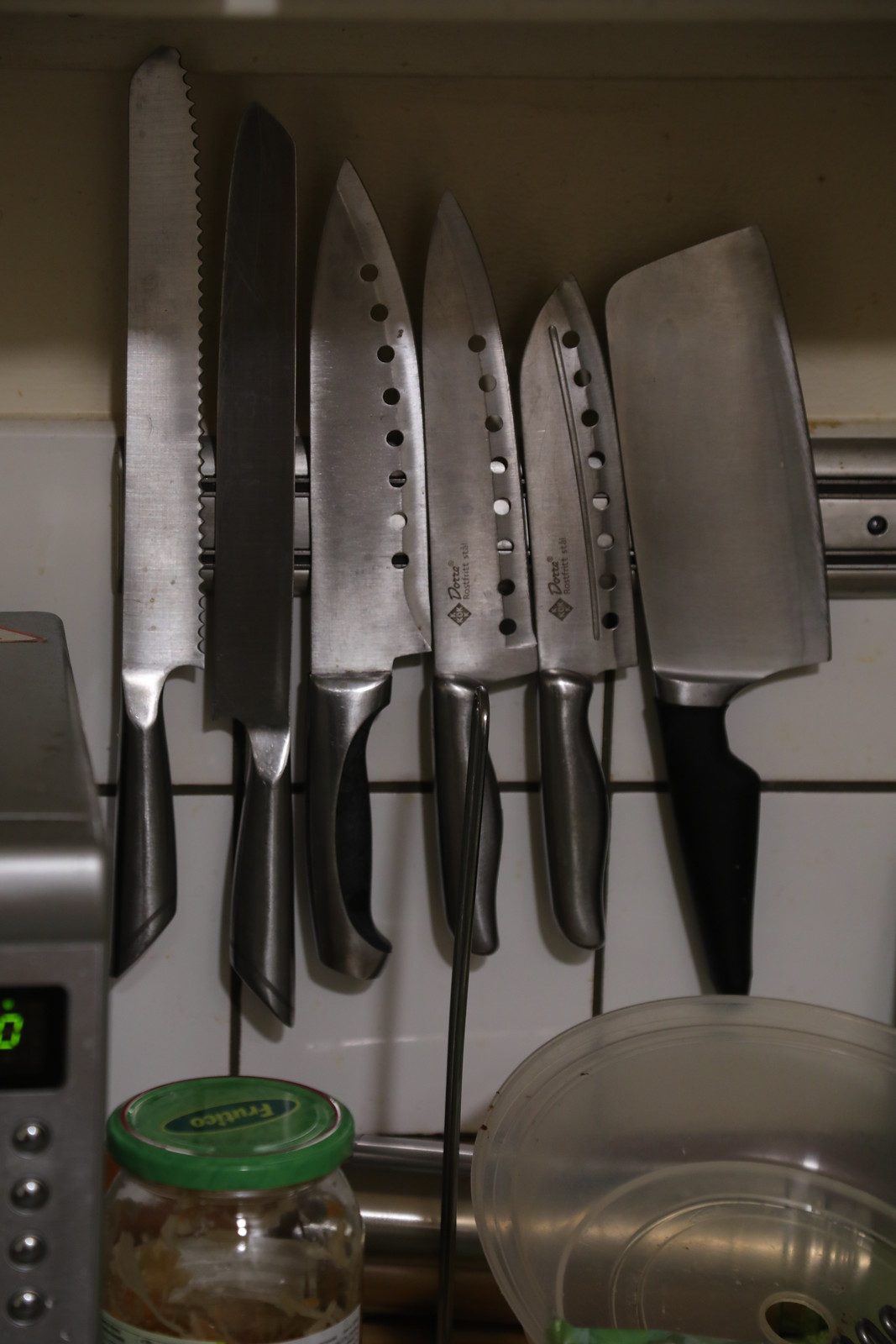The photograph, captured in a kitchen, showcases an organized arrangement of knives and various kitchen items. The backdrop is a white tiled wall onto which six knives are neatly affixed via a metal rack. These knives, all featuring black handles, vary in type and size. From left to right, there is a long serrated knife typically used for bread, followed by a black-bladed knife, two standard chef's knives with a series of small holes along the blades, a smaller chef’s knife, and finally, a large cleaver with a thick rectangular blade. 

In the foreground, a silver microwave sits on a counter showing the number zero on its display. Adjacent to the microwave is a glass jar with a green metal lid, containing what appears to be relish. To its right, there is a translucent plastic bowl. The scene is softly lit, with some shadows cast across the top portion of the knives, adding depth to the image.